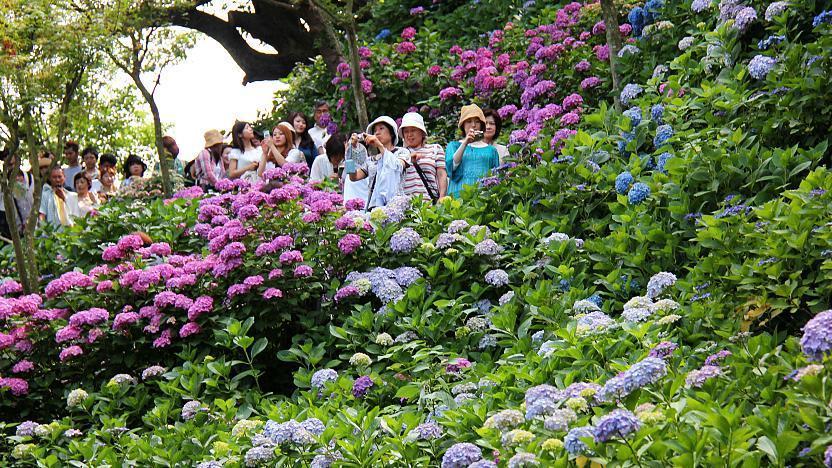This horizontally rectangular outdoor photograph, bathed in natural daylight, captures a picturesque hillside garden teeming with vibrant flowers. The bottom half of the image showcases the lower part of the hill, which is densely populated with tall flowers in various shades of green, blue, light blue, pink, and purple. These flowers, reaching up to the waists of the people in the scene, form a colorful tapestry that extends up the hill.

In the upper left corner, the sky peeks through, along with a scattering of green leaves and tree branches that frame the scene. The photo features a large group of people, predominantly women, standing among the flowers. Most are gathered towards the upper left section of the image, with some holding mobile devices and cameras, intently taking pictures. Many of these individuals are wearing hats, adding a quaint charm to the scene.

The hillside flowers are arranged in clusters: dark blue and purple flowers on the left, transitioning to light blue flowers towards the middle, which then cascade to the right. Above these, more flowers continue up the hill, creating a layered effect of natural beauty. Tiny trees punctuate the landscape, some standing before and behind the group of people.

At the top center-right, a larger tree stretches its branches over the scene. Behind the flower-admiring crowd, the hillside continues its ascent, blanketed with more colorful blooms and eventually blending into the open, light-colored sky in the distance. This serene and enchanting landscape is a harmonious blend of nature's splendor and human appreciation.